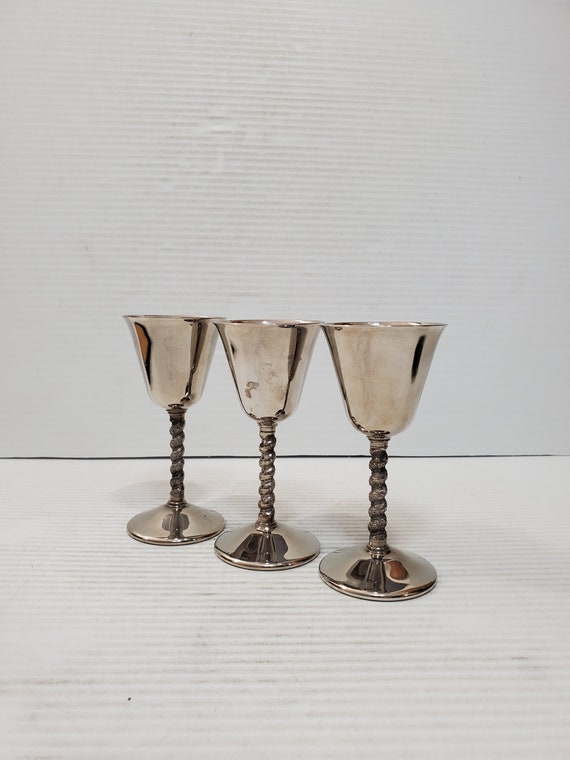This photograph captures a simple, elegant arrangement of three identical goblets, crafted from a shiny, predominantly silver metal with a subtle golden tint. They are positioned diagonally in close proximity on a surface that appears to be white cardboard, situated against a matching white backdrop. The goblets' stems feature a decorative, twisted spiral design, providing a textured contrast to their otherwise smooth, fluted rims. The tops of the goblets flare out, giving them a wider opening compared to their narrower bases. The image is devoid of text and other distractions, placing full emphasis on the medieval-style goblets, which are illuminated by bright, artificial lighting.